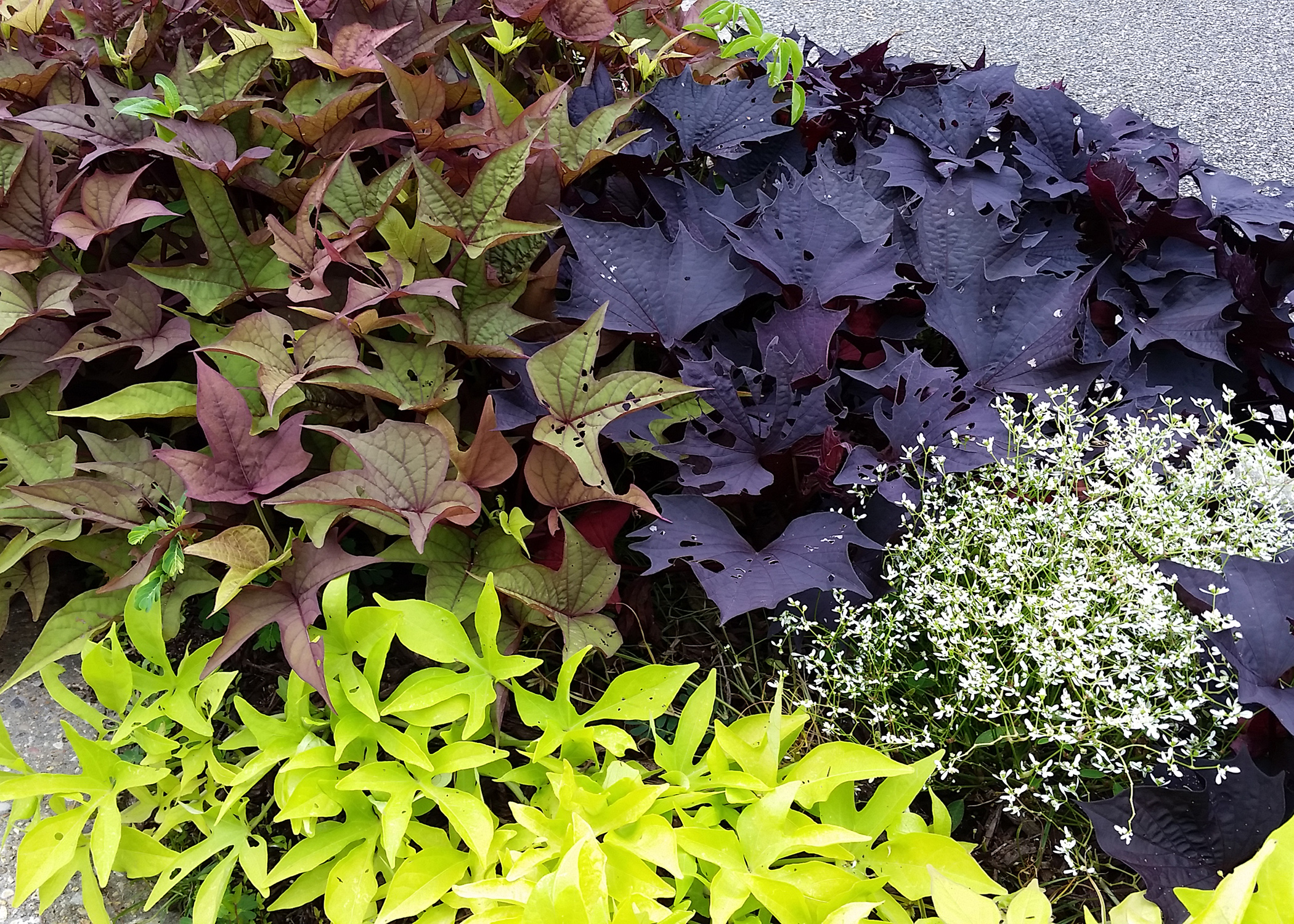This photograph captures a diverse array of outdoor plants, seemingly arranged in a natural environment. On the far upper left, a plant displays broad leaves with a striking blend of green and red, resembling a star pattern. To the right, towards the upper center, there's a plant with large, dark purple leaves, almost oak-like in their shape. Dominating the bottom of the image, a bright yellowish-green plant spans from left to right, its five-pronged leaves, also broad and star-shaped, adding a vivid contrast. Nestled in the bottom right and extending slightly upwards, small white flowers with delicate green leaves offer a dainty touch to the scene. Additionally, there's a patch of green grass with white-topped flowers emerging from the right middle. The upper right corner reveals a bit of ground covered in a white and gray gravel-like texture, providing a subtle backdrop to this botanical assortment.